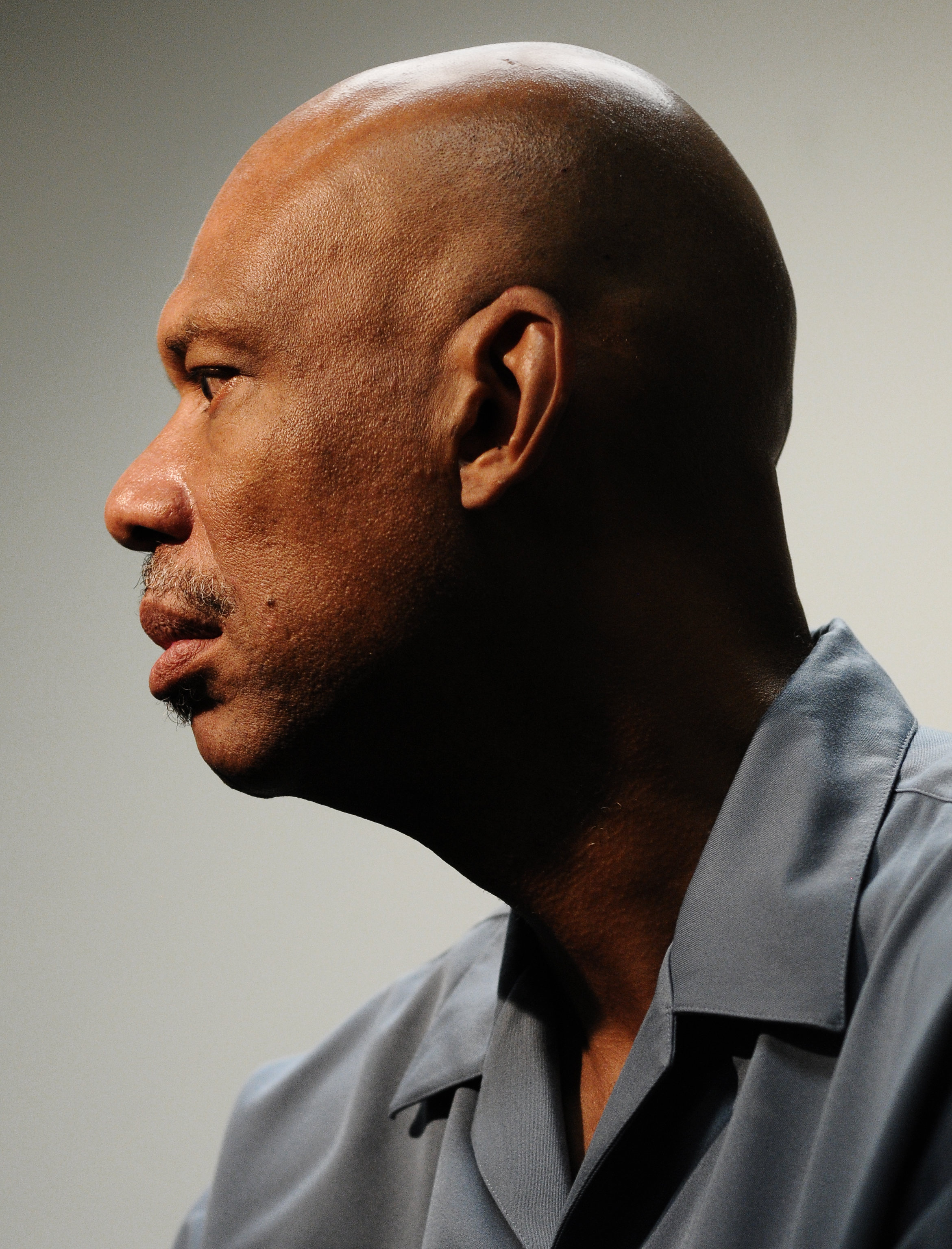This photograph captures a man, prominently positioned, almost filling the entire vertical frame. His head occupies the upper center part of the image, and he is facing slightly to the left. The background is a light gray wall. He is attired in a collared gray shirt that extends off the image at the chest level. He has a light brown complexion, a shaved head, and his black mustache, speckled with white, is complemented by a small patch of hair beneath his lower lip. His dark, slightly bloodshot left eye, the only eye visible, looks downward, contributing to a puzzled expression on his face. Notably, he has a unique mole on the left side of his face, near his mustache, and an oddly shaped left ear situated next to his bald head, reminiscent of Kareem Abdul-Jabbar.